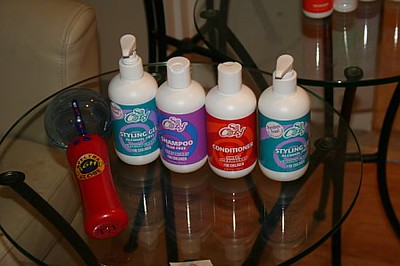The image features a cozy interior scene with a white backdrop and a beige leather chair positioned to the left. The setting includes a brownish-red hardwood floor and showcases two glass-topped tables with black steel legs arranged side by side. The most prominent table holds four labeled hair product bottles. Two bottles feature pump tops—one is emblazoned with "So Cold Styling Gel" in turquoise with lavender accents, and another green one also labeled as styling gel. The remaining two bottles, with flip-top openings, are a shampoo with a dark purple and blue label and a conditioner with a white and red label adorned with lighter red swirls. Adjacent to these bottles, there is a red-handled device featuring a clear acrylic ball at its top and a black and gold sticker, potentially a toy that lights up. The glass surface of the table reflects the bottles clearly, enhancing the organized setting. The other table provides a partial view of similar hair product bottles, maintaining the thematic continuity of the scene. The arrangement of elements and the details of the products create a functional yet aesthetically pleasing environment.